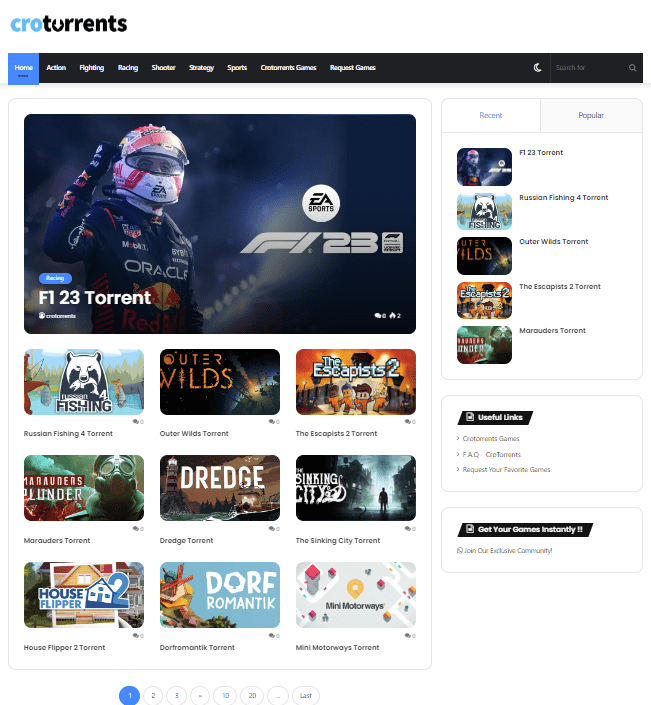The website displays the title "CRO Torrance" with "CRO" in blue and "Torrance" in black, set against a black top navigation bar. The navigation menu includes options such as Home, Action, Fighting, Racing, Shooter, Strategy, Sports, and Request Games. The main image prominently features a motorcycle rider in a black outfit and helmet under the title "F1-23 Torrance" alongside the EA Sports logo. Below this, smaller thumbnails display various game titles including Fishing, Outer Wilds, The Escapes 2, Something Plunder, Dredge, The Sinking City, House Flipper, Dorf Romantic, and Mini Motorways Torrance.

On the right-hand side of the page, a section labeled "Recent and Popular" lists titles such as F1 Torrance, Russian Fission, Outer Winds Torrance, The Escapist Torrance, and a title that seems to be Morrader's or similar. Additionally, there is a "Useful Links" section which includes Frequent Asked Questions, Request Your Favorite Games, Crota Currents Games, and Get Your Games Instantly, offering further engagement options for users.